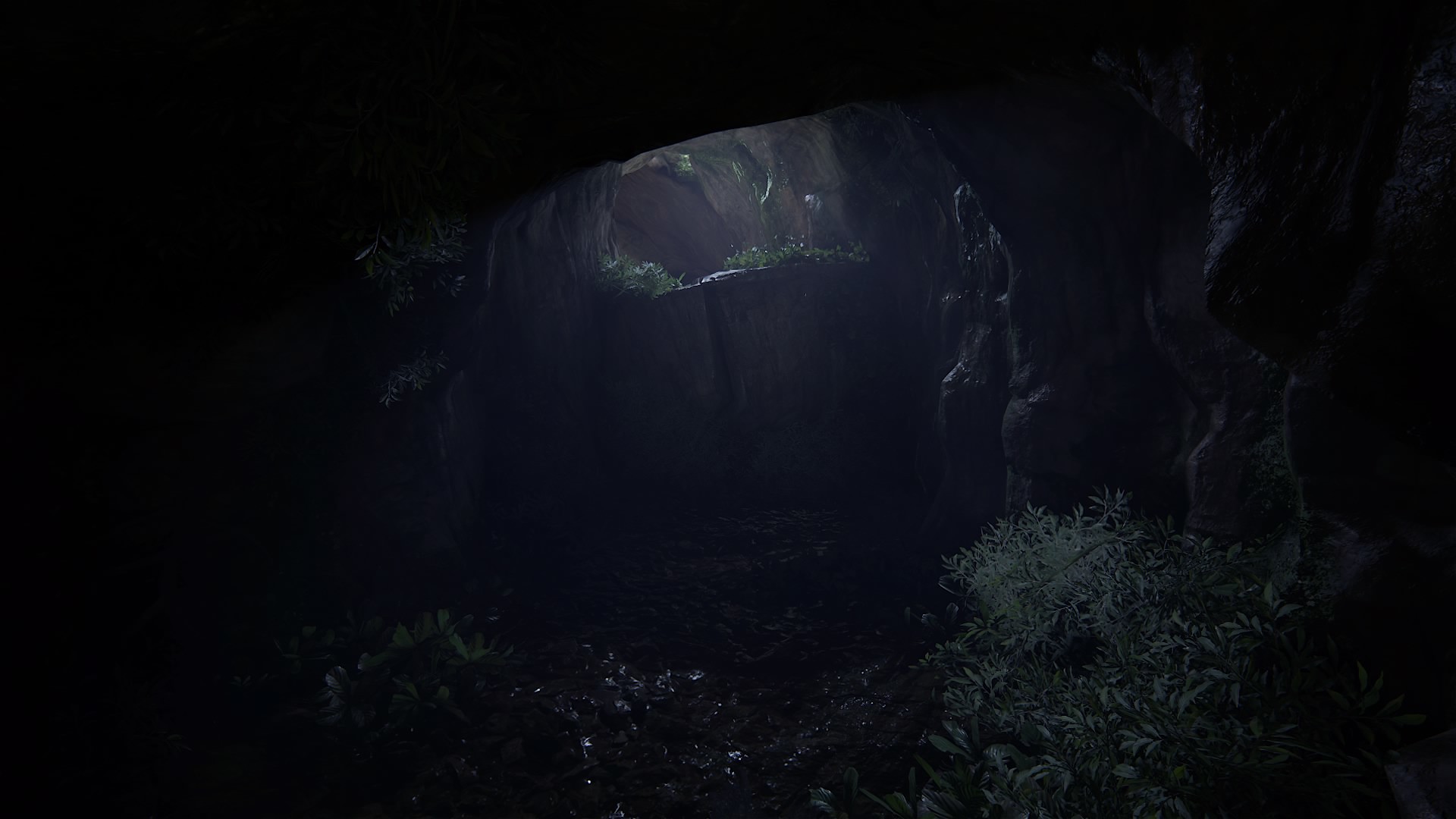This is a dark and moody photograph capturing the interior of a cave with a small, circular opening at the center-top of the image, where sunlight beams through like a shaft of light, illuminating parts of the scene. The cave's entrance is surrounded by rough, rocky terrain with both wet and dry stones. Green and white leafy plants are scattered throughout, adding texture and life to the otherwise stark environment. Notably, there are two stone formations in the lower part of the image that resemble carved legs and feet, creating the impression of a human statue guarding the cave's entrance. Vegetation is present around the circumference of the opening, and a small bush can be seen on the right. The interplay of light and shadows reveals depths within the cave, enhancing its mystique and rugged natural beauty.